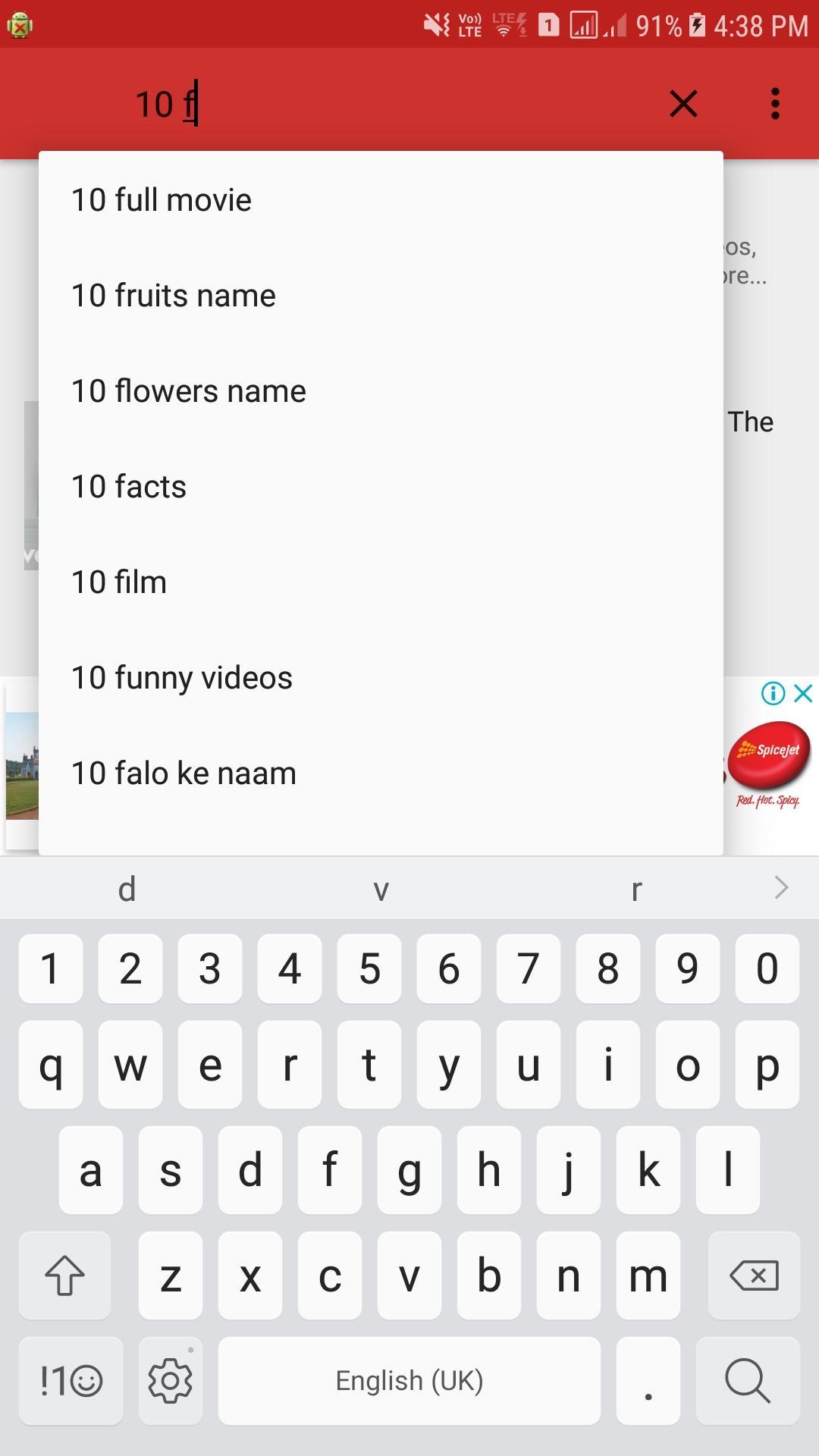A detailed screenshot from an Android smartphone reveals the intricacies of a user interaction within an unspecified app. At the top, a red bar houses a text box where the user has typed "10 F". Below this, a dropdown menu appears, providing predictive text suggestions such as "ten full movie", "ten fruits name", "ten flowers name", "ten facts", "ten film", "ten funny videos", "ten follow key nom" - the latter in an unidentified language. This dropdown obscures the app's content, making it impossible to determine its purpose or functionality. 

In the upper left corner of the status bar, an icon of an Android mascot with an X on its torso indicates an issue. The phone is set to silent mode with vibrations enabled, and it is currently connected to an LTE network with three bars of signal strength. The battery is charged at 91%, and the time displayed is 4:38 p.m.

At the bottom of the screen, the on-screen keyboard is visible due to the ongoing typing activity. Partially obscured text behind the dropdown hints at incomplete sentences; one line ends with "OS,", another with "RE...", and another features "the". 

In the lower left corner, a small fragment of a photograph shows a blue sky, green grass, and a building, though the subject remains indistinguishable. On the right side of the screen, an advertisement banner features an information icon inside a circle and an X to close the ad. The ad itself shows a rough red oval shape branded with "Spice Jet" and the tagline "fast, hot, spicy" below it.